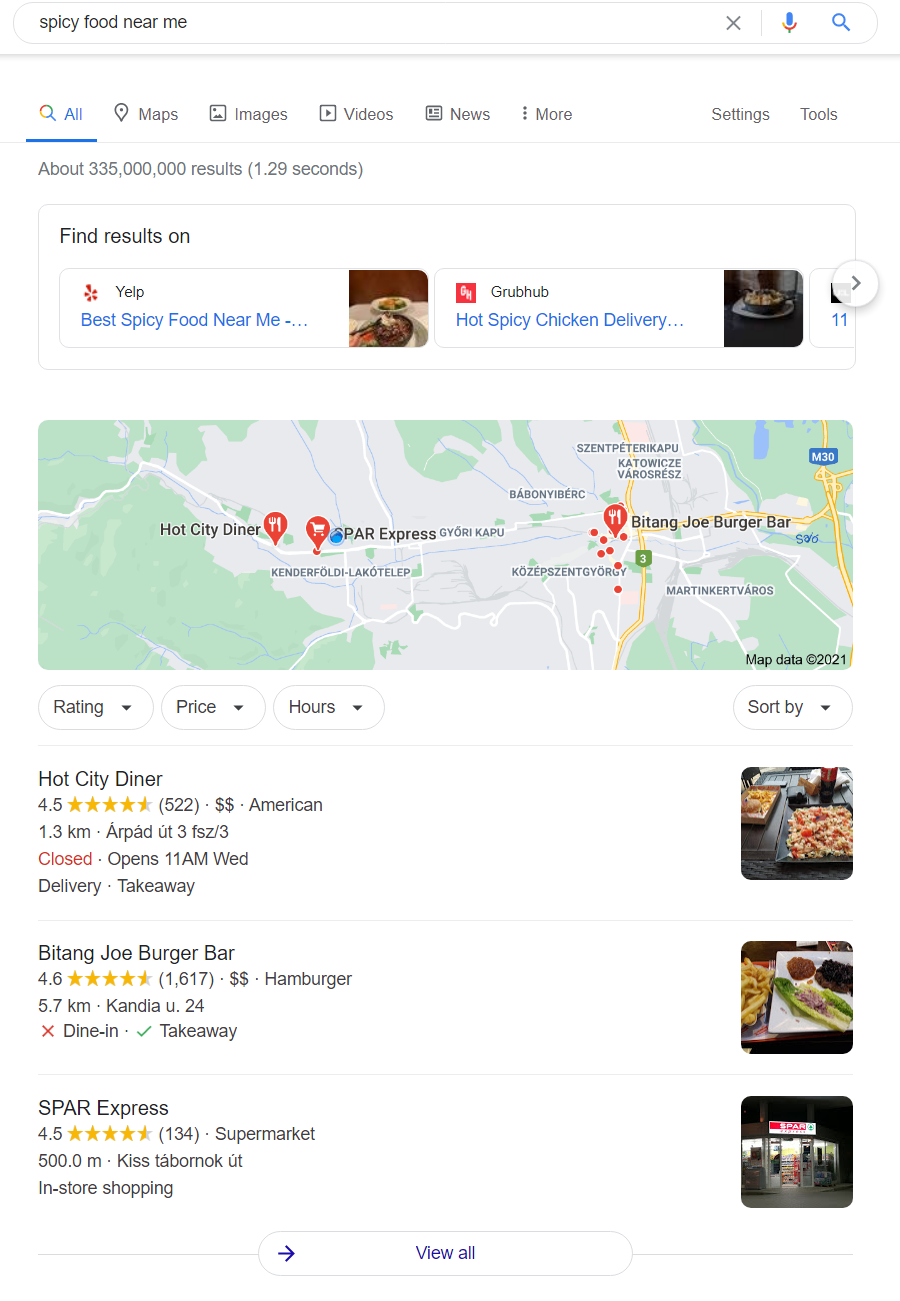The image captures the results of a Google search for "black spicy food near me." At the top of the screen, the search query is displayed in the search box, and the search yielded approximately 335 million results in just 1.29 seconds. Immediately below the search box, there's a small section with links to different food service platforms, including "Find results on Yelp" and "Grubhub." Yelp suggests "Best Spicy Food Near Me," while Grubhub features "Hot Spicy Chicken Delivery."

Below this section, a map highlights three prominent search results in the vicinity:

1. **Hot City Diner:** Rated 4.5 out of 5 stars, this American diner is positioned on the far left of the map.
2. **Betong Joe Burger Bar:** This hamburger place, boasting a rating of 4.6 out of 5 stars, is located on the far right of the map.
3. **Spa Express:** A supermarket rated 4.5 out of 5 stars, situated in the middle of the three highlighted locations.

Each of these establishments is marked on the map, providing a visual representation of their relative locations.